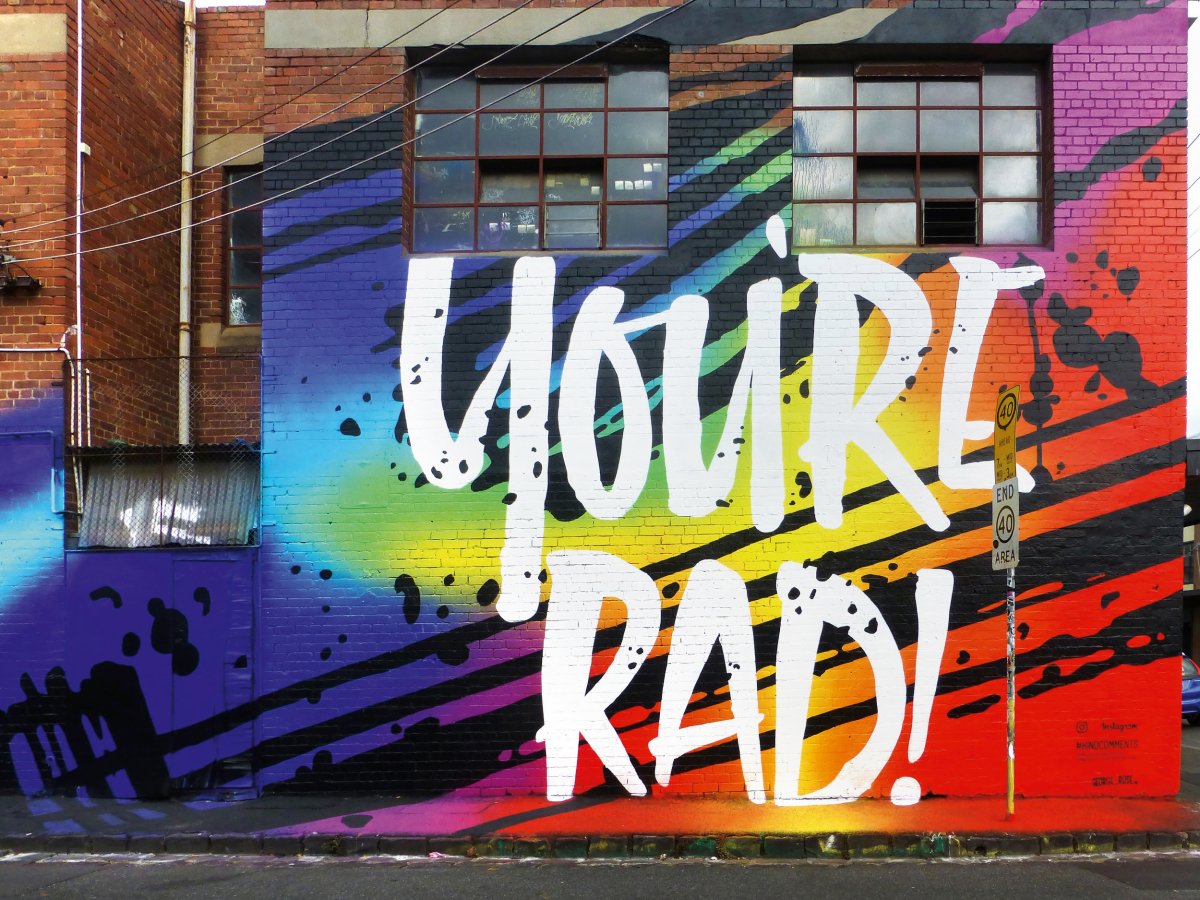The image depicts a red brick building, possibly an industrial warehouse, captured in a landscape orientation. The building features two large, multi-paned windows at the top, each with 16 panes. The right side includes a mile-per-hour street sign indicating a speed limit of 40. The left half of the brick wall is adorned with a vibrant, colorful mural that appears to be either spray-painted or digitally added. This mural showcases an array of colors transitioning from violet and dark blues on the left, through greens and yellows in the center, to reds and oranges on the right. Black abstract streaks and splotches add texture to the mural. In bold, white handwritten letters at the center, the mural enthusiastically proclaims, "You're rad!"